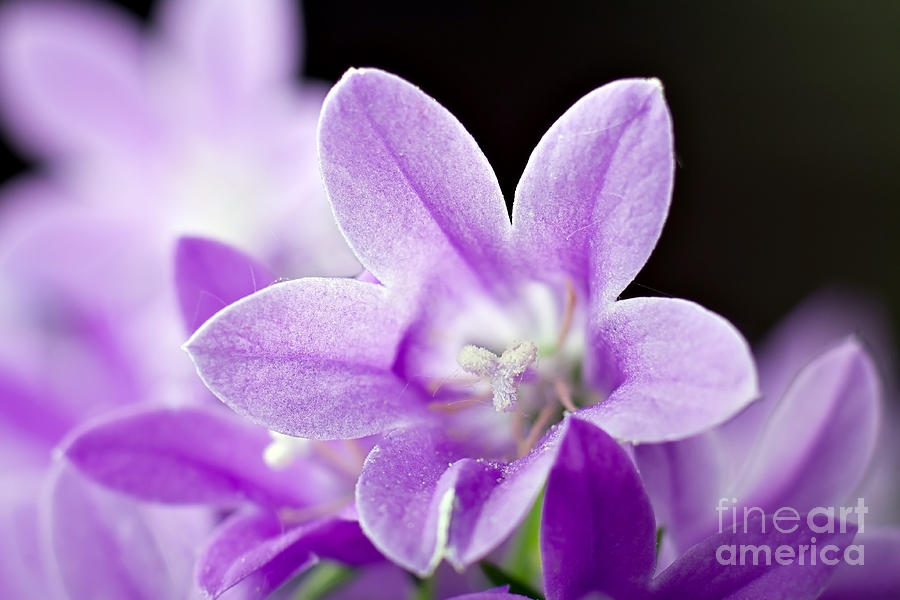This close-up, detailed photograph captures an exquisite arrangement of purple flowers set against a stark black background. The most prominent flower, positioned in the forefront, features five soft, oval-shaped petals surrounding a white, three-pronged stamen accented with delicate pink strands. Its pale purple hue, laced with subtle white hints, gives it a grainy and slightly fuzzy texture. Behind it, partially visible are more purple flowers, some slightly darker and others similarly colored, with their edges and shapes blurred to emphasize the sharpness of the primary flower. A hint of green stems faintly peeks through, adding depth to the composition. The photograph is intricately detailed, showcasing the pollen, stamens, and the floral structure with striking clarity. In the lower right-hand corner, the text "Fine Art America" is subtly inscribed in transparent white, marking the artwork’s authenticity.